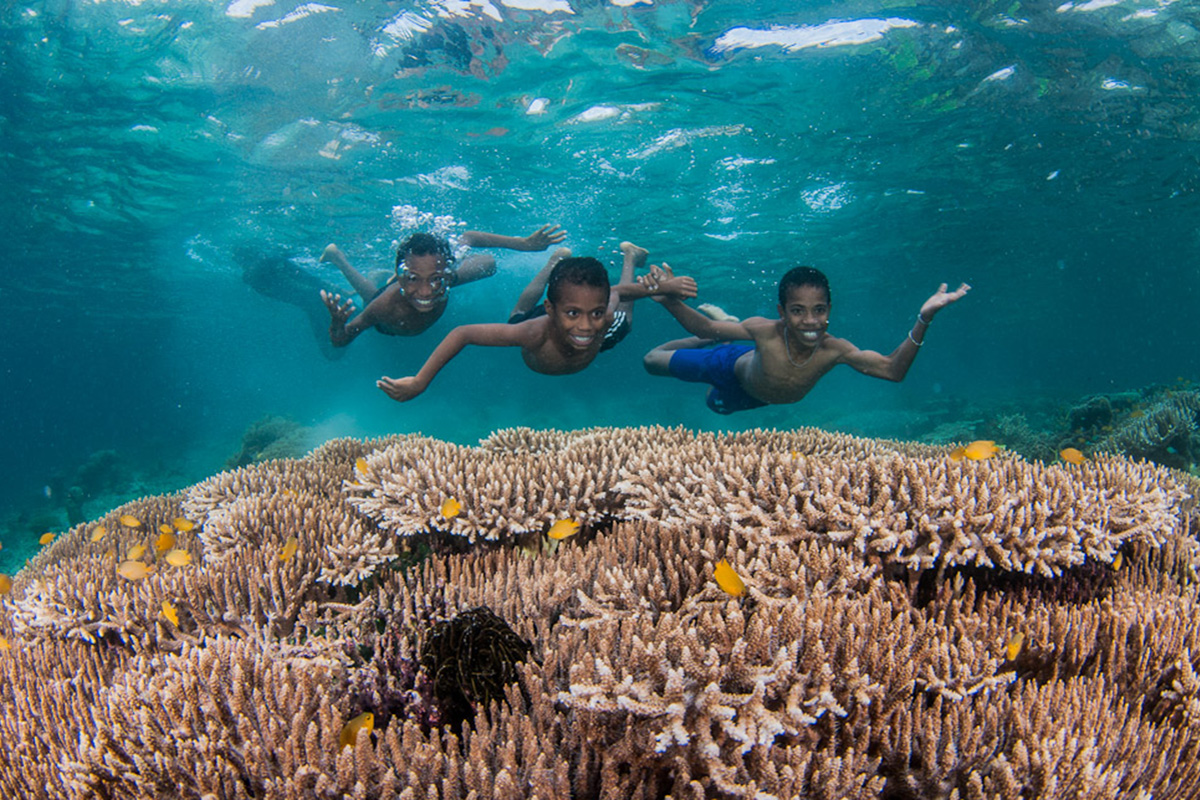This underwater color photograph captures a close-up scene of three shirtless young boys swimming above a coral reef. The water is clear and blue, with light shining through from the surface and creating a ruffled effect. The boys appear to be close in age, possibly triplets or brothers, all with dark hair. The boy on the left is smiling and has his hand up in the air, creating bubbles around him, while his other arm is swimming. The middle boy is wearing black trunks with white lettering and has both arms underwater. To the right, the boy in blue trunks is wearing two silver bracelets and holding the middle boy's hand. Below them, the bottom half of the photograph is filled with brown coral with beige tips, interspersed with small orange and yellow fish. There's also a black hole-like feature in the center of the coral, and some rocks are visible to the right of the frame. The coral transitions from a tannish white to a greenish hue as it moves into the background.